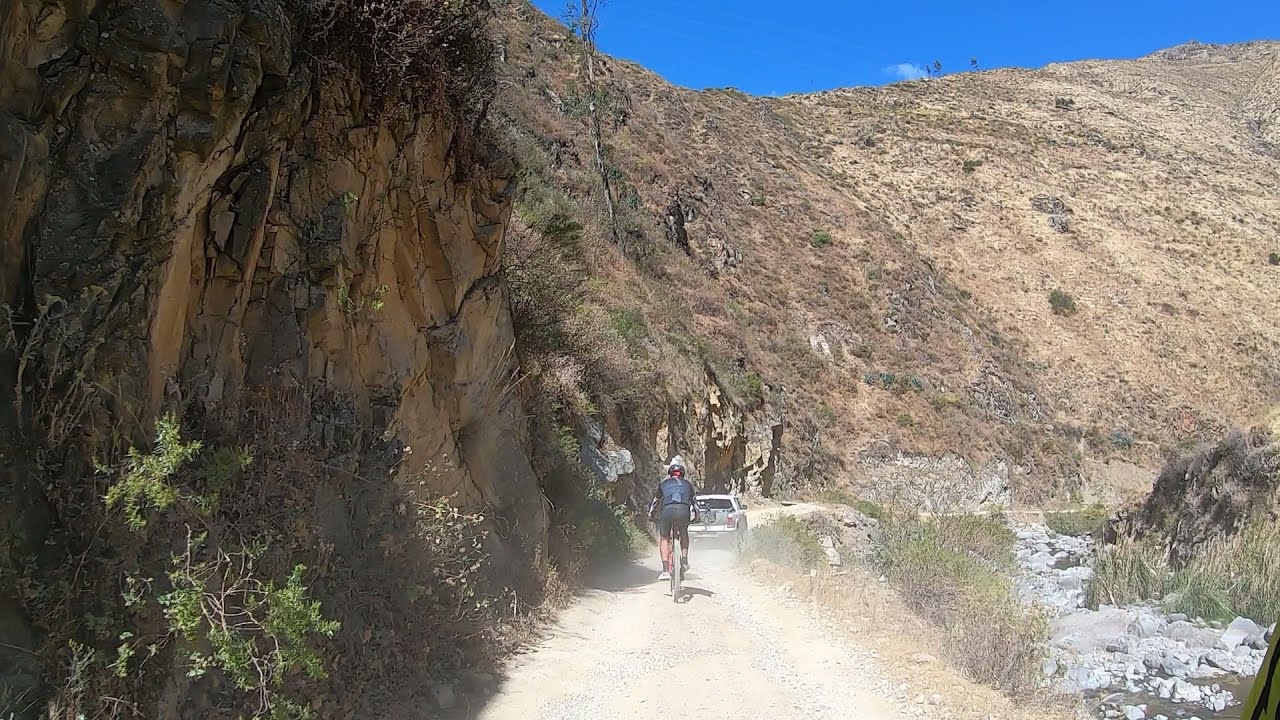In the image, a dirt road cuts through a rugged outdoor landscape dominated by a towering, rocky cliff that extends across most of the frame. A white truck drives along the dusty path, closely followed by a cyclist wearing a blue shirt, black shorts, and a red helmet. To the left of the road, the cliffside is a mixture of stone and dirt, adorned with patches of grass and sparse, small trees. On the right, the terrain descends into what appears to be a rocky creek bed, with tall green grasses and brown rocks scattered throughout. The sky above is clear and blue with a few wisps of cloud, suggesting a sunny day. Light shrubbery and weeds grow near both the cliff and the creek bed, adding to the dry, rugged feel of the scene. The road itself is wide enough for vehicles, making it ideal for off-road biking.